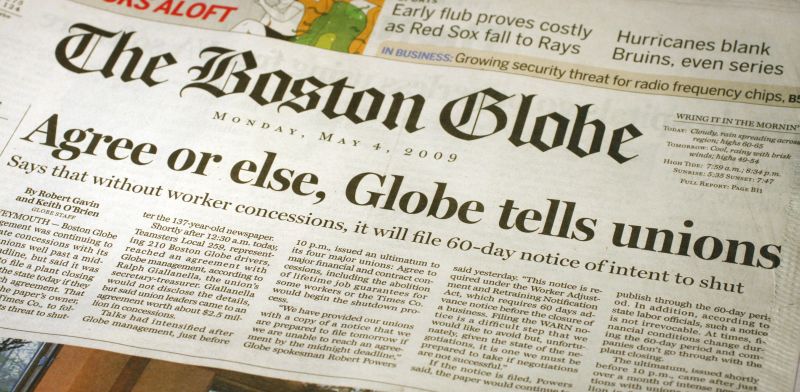This is a photograph of the front page of the Boston Globe newspaper dated Monday, May 4th, 2009. The image shows the newspaper placed on a surface, photographed at an angle, and only the upper portion of the page is visible. The headline reads prominently, "Agree or Else, Globe Tells Unions," with a sub-headline stating, "Says that without worker concessions, it will file 60-day notice of intent to shut." In addition to the main headline, above the masthead are two news briefs: "Early Flub Proves Costly as Red Sox Fall to Rays," and "Hurricanes Blank Bruins Even Series," along with a smaller item in the business section titled, "Growing Security Threat for Radio Frequency Chips." The detailed font used for the Boston Globe title and the clear date emphasize the newspaper's branding and the specific day of publication.